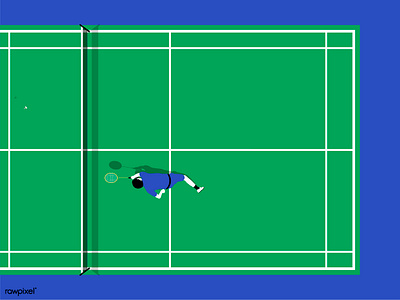This image, seemingly a still from a simple tennis video game, is captured from a bird's eye view. The background surrounding the green tennis court is a medium bright blue, highlighting the court’s vibrant green surface with neatly defined white lines. In the bottom left corner, tiny black letters spell out "now pixel" or "row pixel." 

The scene features a tennis player with white skin, black hair, and dressed in a blue uniform consisting of a shirt and shorts. He sports white sneakers with black socks reaching up to his calves. Positioned mid-hit, the player's black-shadowed form reveals a detailed yellow tennis racket with a black grip and a green metal rod. A small white tennis ball is visible in the top left corner against the blue backdrop. All these elements together create a clean, digital, and somewhat simplistic visual impression characteristic of vintage or basic tennis video games.